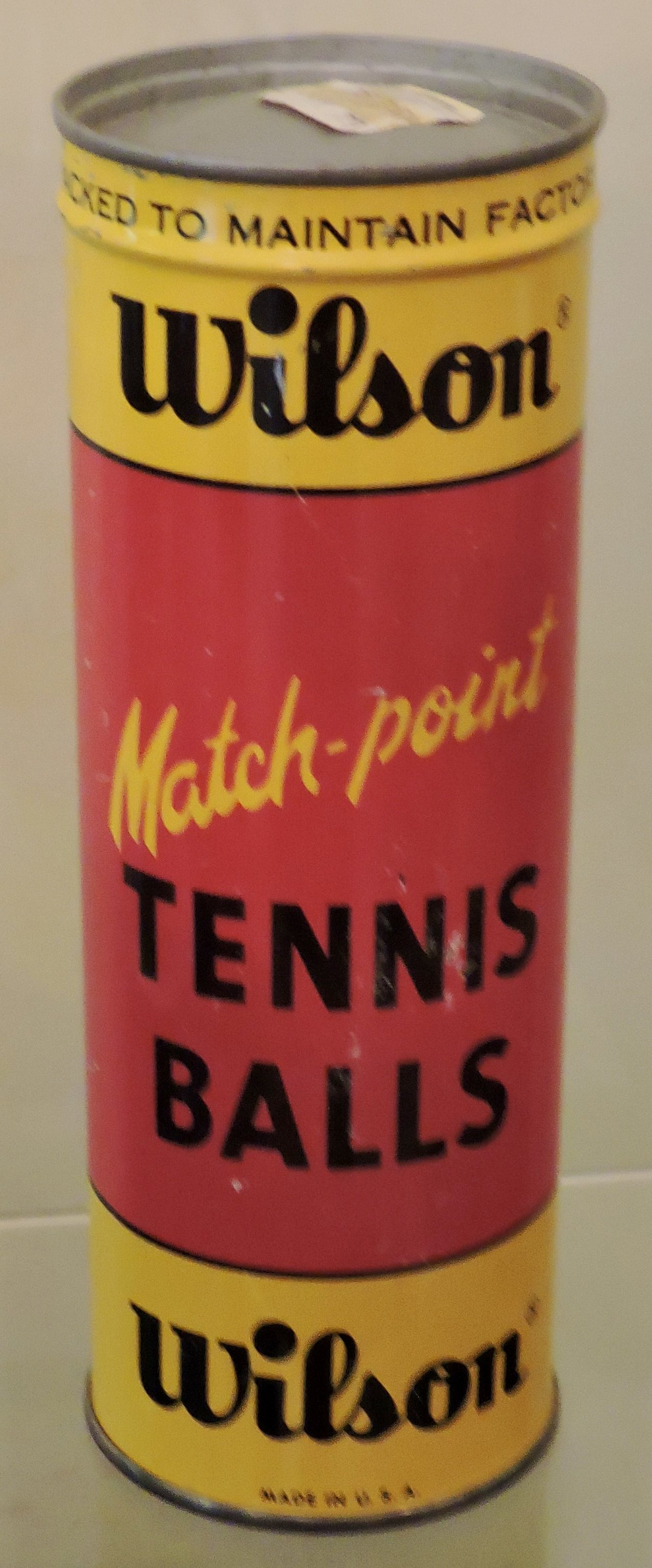This image features a vintage can of tennis balls, captured with a slightly grainy, old-fashioned quality. The cylindrical can appears to be made of metal, although the exact material is uncertain. The can's design is striking, with a vibrant yellow and red color scheme adorned with black lettering. The top of the can features a pop-top lid in gray. Prominently displayed on the can is the brand name "Wilson," and the text "Match Point Tennis Balls" is also visible. A second "Wilson" is printed at the bottom of the can along with the phrase "Made in the USA." The bottom section of the can is a distinct gray, and the can appears to be unopened, preserving its contents in their original condition.